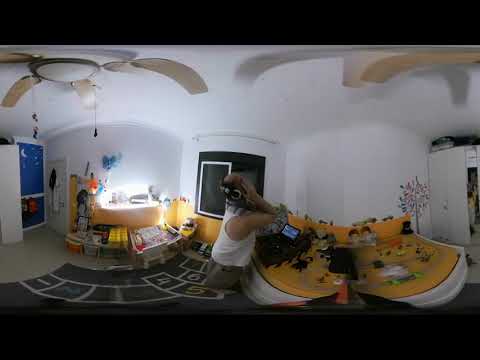The image depicts the interior of a room, possibly a children's playroom, characterized by its white walls and ceiling. Two ceiling fans, each with a beige and white light bulb at the center, are mounted on the ceiling. The fan on the left side has visibly bent, light brown blades, while the fan on the right is partially visible with only one blade in view.

The left side of the room features a blue cabinet, situated next to an assortment of toy boxes and a small red children's desk with a white chair. In front of the toy box lies a black mat with a white box pattern and numbers, resembling a hopscotch design. The floor appears to be tiled with a child's play carpet overlaying it.

On the right side of the image is a yellow playstation with white sides. A person is at the center of the image, leaning against the counter of the playstation. This individual, wearing a white tank top, brown bottoms, and a black headset, has their hands over their eyes as if looking up at the ceiling.

The photograph itself is a smaller, horizontally aligned rectangle framed by thick black borders at the top and bottom. The overall scene is colorful, incorporating shades of white, blue, yellow, tan, black, and gray.